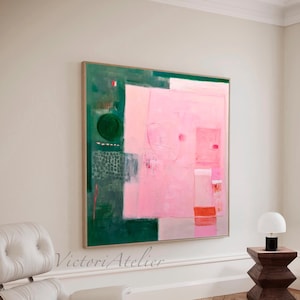The image showcases an elegant wall, likely in an art gallery or a sophisticated modern home, painted in a light beige color with white crown and other moldings. A striking square painting is the focal point, featuring a modern mix of vibrant colors and intricate patterns, predominantly in shades of pink and green, with hints of orange, dark blue, black, and red. These colors create a textured and dynamic composition that may resemble views of a landscape or abstract designs. Below the artwork, the text "Victoria Atelier" is visible, crediting the artist. The setting includes a unique brown lamp with a white bulb positioned to the right, atop a modern table, and a portion of a white chair or sofa is visible at the bottom left corner. The overall neutral tones of the walls and furnishings complement the vivid painting, making it stand out beautifully in the serene and stylish environment.